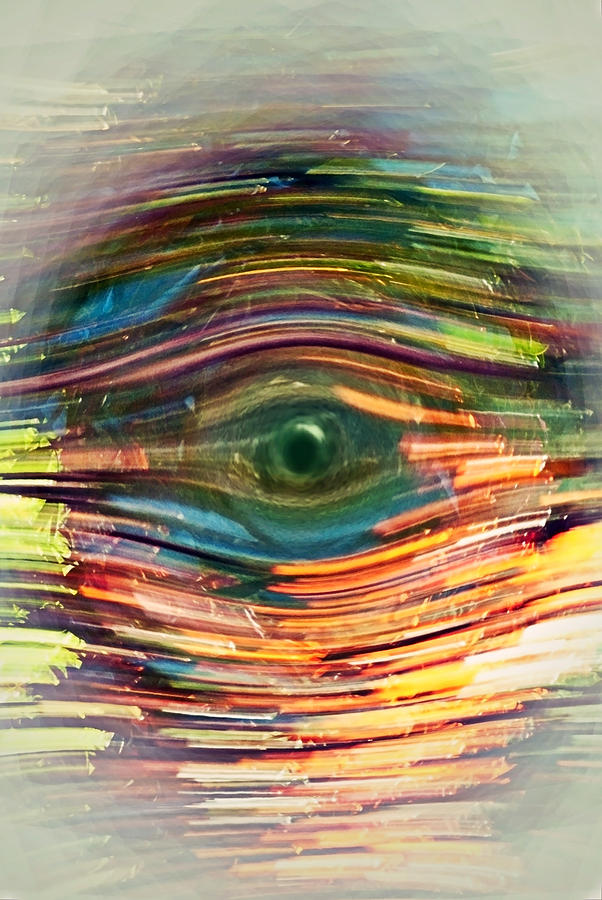A vibrant, abstract image capturing an eye-like form at its center, exuding an enigmatic quality open to interpretation. The central focal point resembles a round, piercing eye, akin to that of a crocodile, surrounded by a full spectrum of vivid colors. Radiating from this “eye” are graceful, curved lines above and below, creating a mesmerizing ripple effect, reminiscent of the disturbance caused when an object is dropped into water. The intensity of the colors is strongest near this central 'eye,' gradually becoming faint and blurred as they move outward, enhancing the sense of depth and movement in the artwork. This intriguing composition invites the viewer to envision looking down into a mysterious, colorful body of water with a captivating eye gazing back.